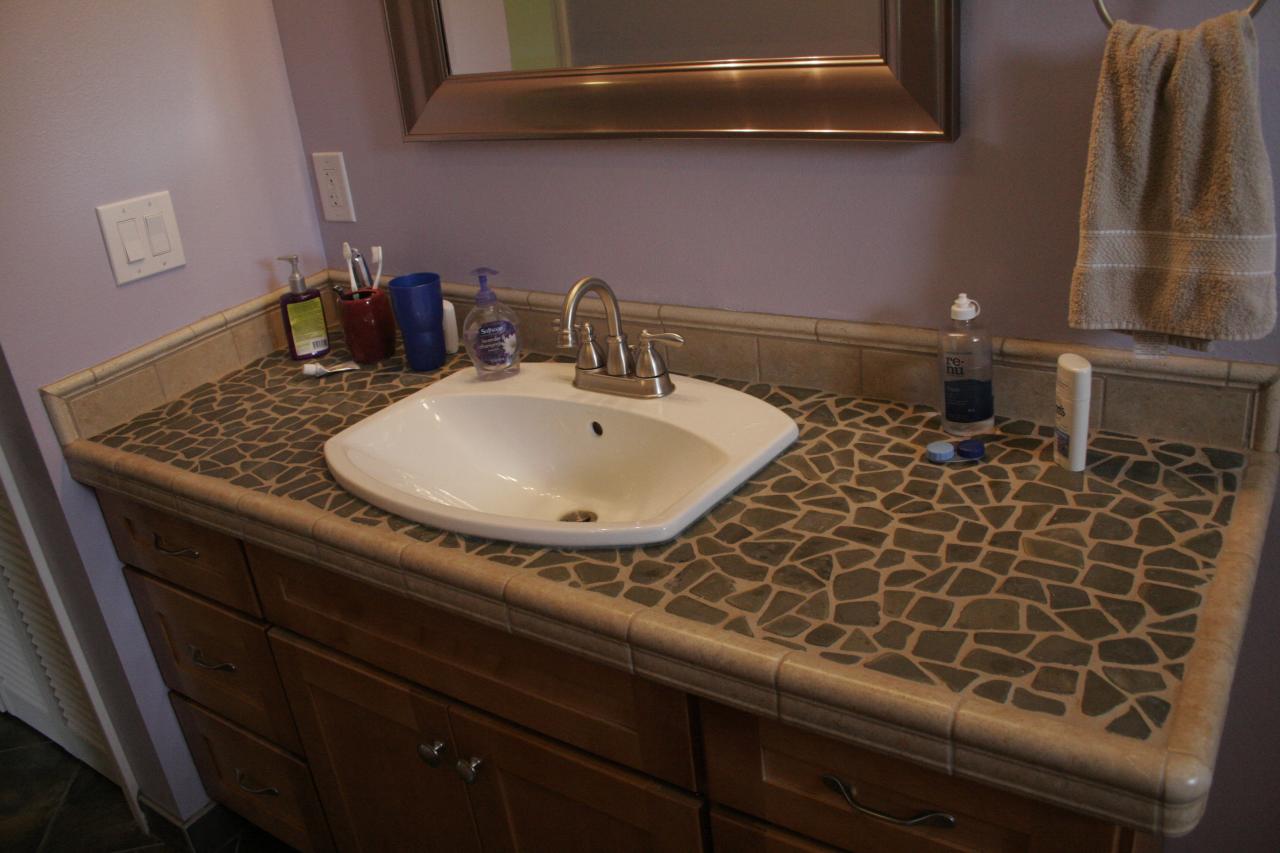The photograph showcases a rectangular-shaped residential bathroom sink area. The serene ambience is set by light lilac purple walls, creating a calming backdrop. The sink's countertop exhibits a rustic charm with small, irregularly shaped gray stones embedded on a tanned surface, adding texture and character. Below, dark brown wooden cabinets with sleek silver-colored knobs accentuate the elegance and provide storage.

The sink itself is a centerpiece with its rectangular shape, featuring a gracefully curved faucet with dual handles for temperature control. Positioned at the back end of the sink, a small round clear plastic bottle with a purple label and a purple pump sits ready for use, likely containing soap or lotion.

On the top right corner of the image, a brushed metal towel ring affixed to the wall holds a neat brown hand towel, easily accessible for drying hands. Directly beneath this towel ring, a small rectangular deodorant stick with a white cap and a blue and white label is positioned, reflecting the practical organization of personal hygiene items in this thoughtfully designed bathroom space.